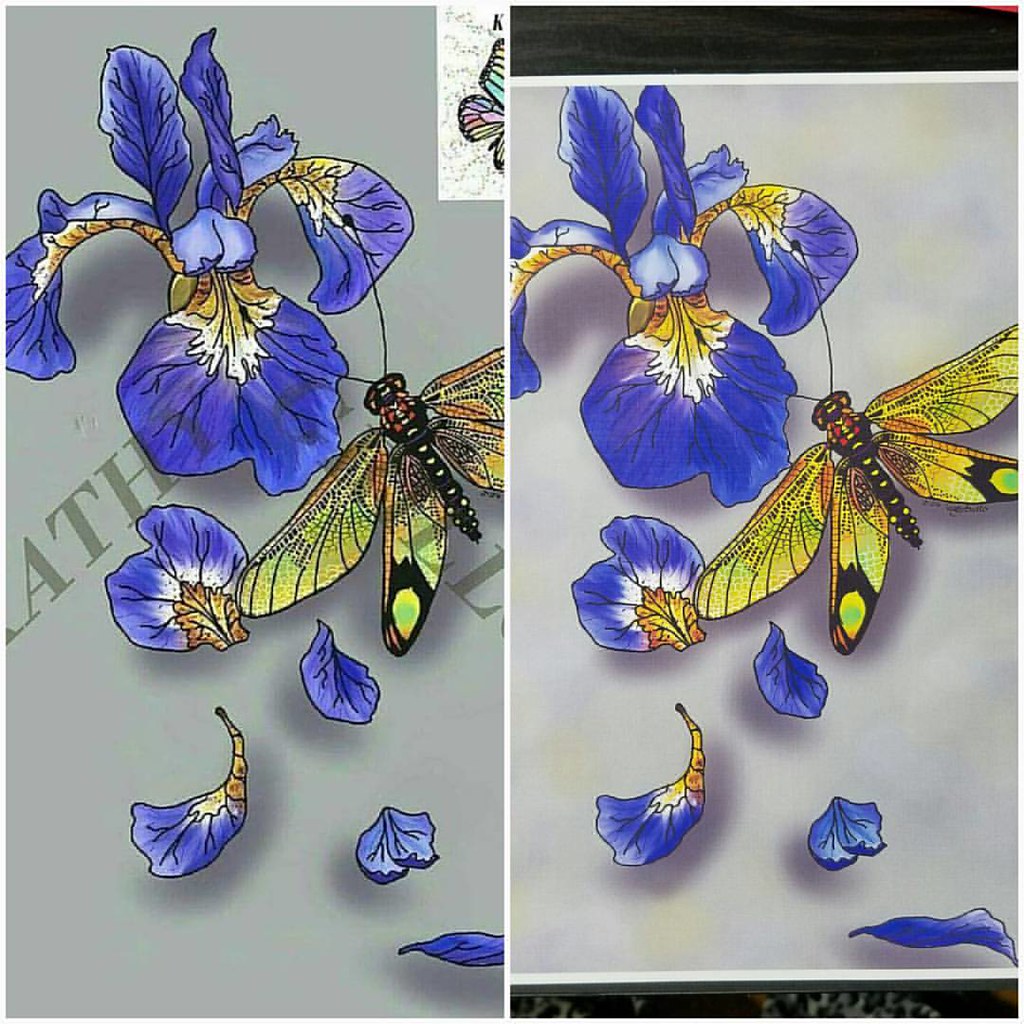In this side-by-side image comparison, the left photograph showcases a drawn or painted depiction of a vivid blue and yellow flower with some petals gracefully falling against a gray background. Adjacent to the flower, a striking yellow and black dragonfly is illustrated in mid-flight. Diagonally across this illustration, a faint text is inscribed, although its content is not distinctly legible. In contrast, the right photograph presents an almost identical scene. However, this version is devoid of the diagonal text and seems slightly zoomed out, revealing the complete borders or edges of the artwork, offering a clearer view of the entire composition.